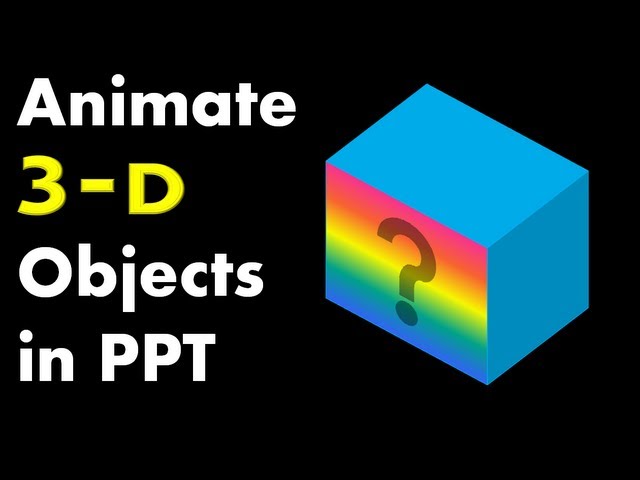The image features a stark black background with the text "Animate 3D Objects in PPT." The words "Animate Objects" and "in PPT" are rendered in white, while "3D" is highlighted in yellow, with a yellow dash between the "3" and "D." Positioned prominently to the right of the text is a blue cube. The front face of this cube displays a vibrant rainbow pattern transitioning from pink to purple and bears a black question mark at its center. There are no other elements or watermarks present, suggesting the image serves as a straightforward advertisement or poster for utilizing 3D objects in PowerPoint (PPT).